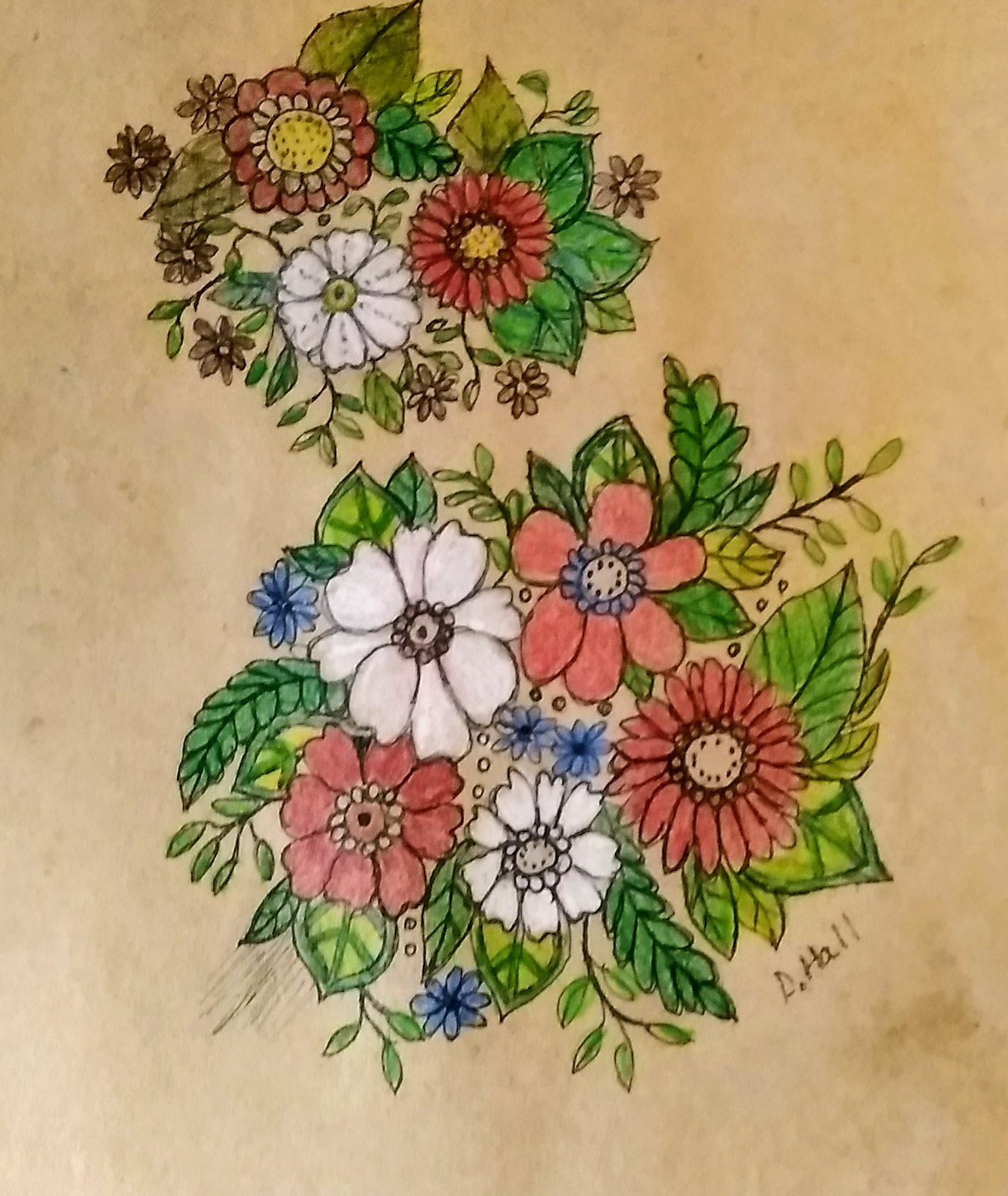This detailed hand-drawn image features an array of meticulously illustrated flowers, each outlined in black pencil to highlight the intricate details of their petals. The artist, D. Hall, has used a variety of colors to bring the flowers to life, including rich shades of purple, vibrant reds, lighter red hues, pristine whites, and tiny brown flowers that form a delicate border around the main blooms. The scene is further enhanced by leaves in varying shades of green, from bright and lively greens to deeper, olive tones. All of this artistry is presented against a warm, tan background, adding a natural, textured feel to the overall composition.